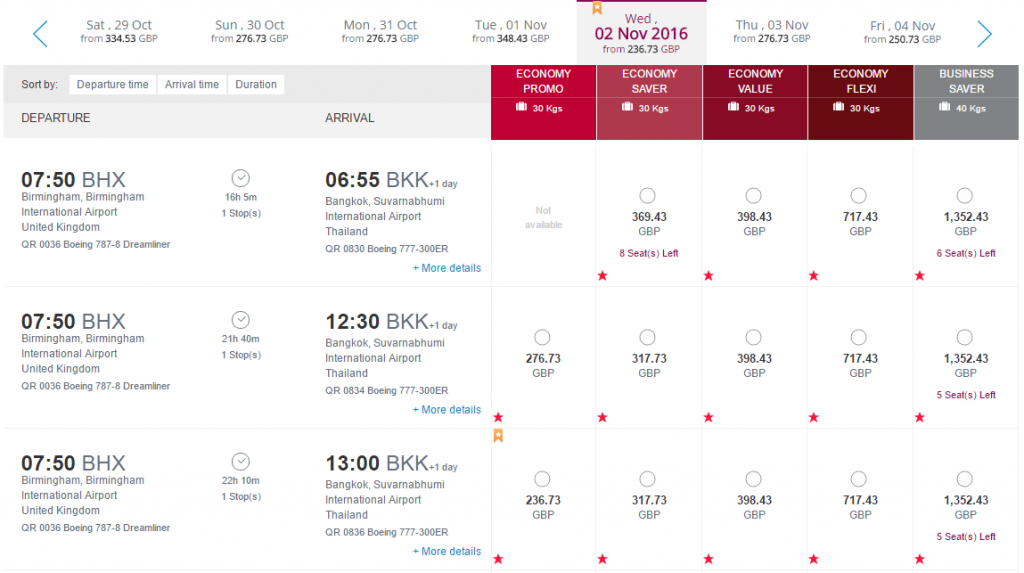The image features a detailed schedule layout with various sections and colored elements. At the top, there is a calendar view with a series of dates starting from Saturday, October 29th, progressing through to Sunday, October 30th, and highlighted is Wednesday, November 2nd, 2016. This particular date is enclosed in a prominent purple box with a darker purple line across it and an orange tag in the upper left corner. The dates extend through to Thursday and Friday. On either side of the calendar display, there are blue arrows pointing left and right.

Below the calendar, a gray box offers sorting options for departure time, arrival time, and duration, leading into detailed information on departures and arrivals. To the right of this section, five distinct color-coded boxes indicate different fare classes: light purple for Economy, deeper purple for Economy Saver, even deeper purple for Economy Value, darker purple for Economy Flex, and gray for Business Saver. 

The background of the image is white, segmented into various boxes containing flight details. The flight identifier "0750BHX" appears multiple times, each accompanied by a small clock icon. Flight identifiers "655BKK," "1230BKK," and "1300BKK" are also displayed. Purple stars are scattered across specific times, such as the area above "1300BKK," where a single purple star is positioned alongside an orange tag with a tiny mark beneath it.